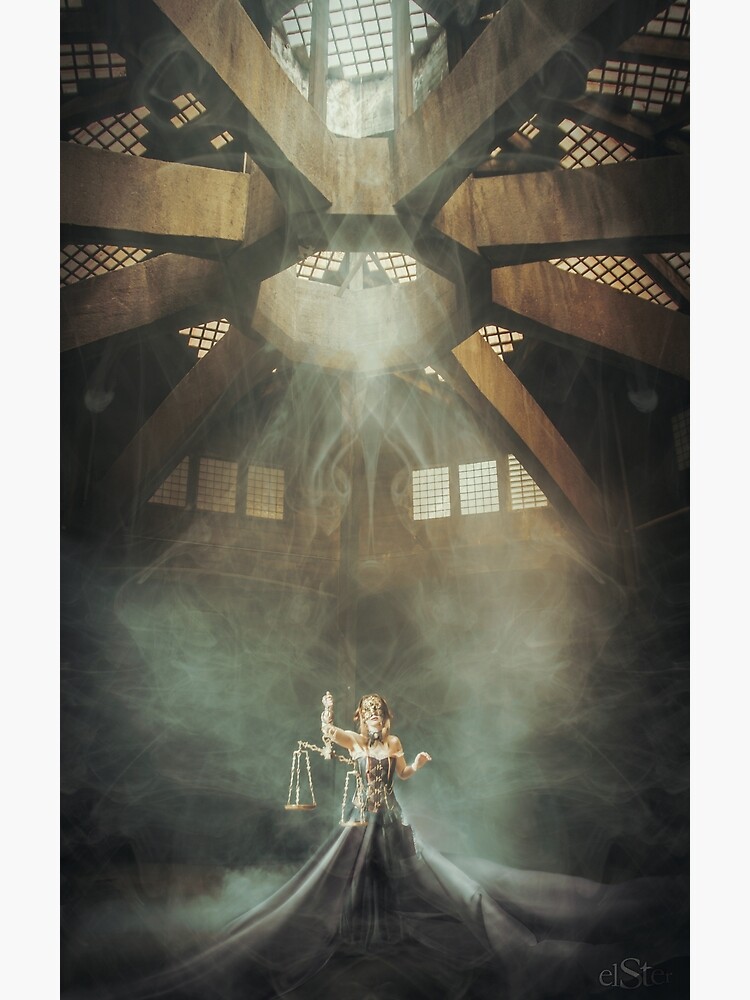In this sophisticated and moody photograph, a woman stands dramatically at the center, enveloped in a strapless, tight-fitting black gown that flows expansively around her. Her dress seamlessly merges with the floor, creating a striking visual effect. She dons a delicate, masquerade-style mask that covers her eyes, adding an air of mystery. In one hand, she holds a pair of golden balancing scales, symbolizing law and justice. The setting is an imposing, circular domed room, characterized by large wooden beams arranged in a sunburst pattern on the ceiling, complemented by a mesh-like grid. The room, shrouded in a smoky haze, exudes an eerie darkness, with light filtering through small windows. This interplay of light and shadow casts the woman in a luminous yet somber glow, enhancing the enigmatic and almost surreal atmosphere of the scene.